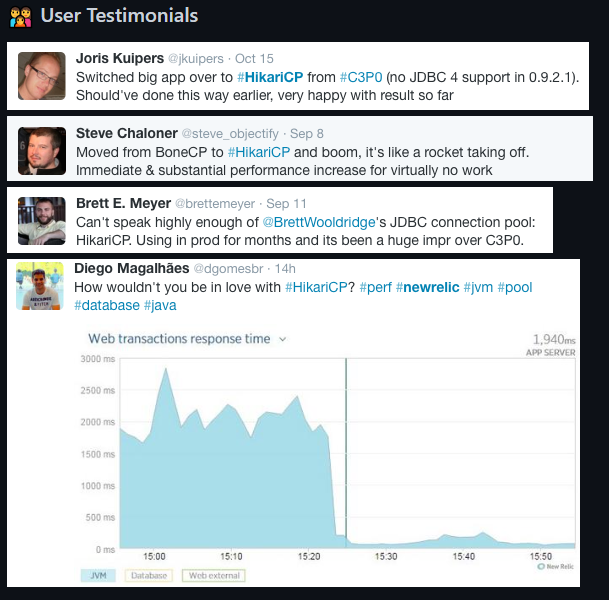**User Testimonials Highlighting the Akari CP Transition**

At the very top of the image, in bold white text against a black background, the word "Testimonials" is prominently displayed. To the left of this text is a picture of a family featuring a mom, dad, and their child. Beneath this header, there are testimonials from three different users, each accompanied by their respective profile pictures and comments.

1. **Joris Culper**:
   - **Profile Image**: A middle-aged man with glasses and a receding hairline.
   - **Date**: October 15
   - **Comment**: "Switched our main app over to the Akari CP from C3P0 (no JDBC support version 0.9.2.1). We should have made this transition much earlier. Very happy with the results so far."

2. **Steve Chandler**:
   - **Profile Image**: [Image not described]
   - **Date**: September 8
   - **Comment**: "Moved from BoneCP to Akari CP, and the change was immediate. It’s like a rocket taking off—substantial performance increase for virtually no effort."

3. **Brad Meyers**:
   - **Profile Image**: Brad is sitting with his elbows on his knees.
   - **Date**: September 11
   - **Comment**: "Akari CP has been a huge improvement over C3P0. We've been using it in production for months and can't speak highly enough of its performance."

4. **Diago Mahalas**:
   - **Profile Image**: [Image not described]
   - **Date**: 14 hours ago
   - **Comment**: "Who wouldn’t be in love with Akari CP? Our New Relic JVM pool database metrics have significantly improved."

At the bottom of the image, there is a detailed line graph showing web transaction response times ranging from 0 milliseconds up to 3,000 milliseconds. The X-axis is labeled from 1515 to 1550. The graph features multiple data series, with the JVM series highlighted in blue. There are also buttons for viewing database and web external metrics.